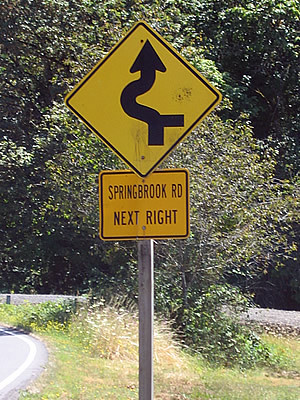The image captures a sunny outdoor scene featuring a significant road sign mounted on a gray metal pole. The primary sign indicates an upcoming intersection on a curving road, depicted with a right-angle symbol at the bottom — showcasing a road that continues straight with another road intersecting from the right. The curve depicted bends to the left, with an arrow pointing straight ahead. Below this, a secondary sign provides additional information, stating "Springbrook Road next right." The background includes a large bush and several trees, highlighting the greenery of the area. The white line visible at the bottom left suggests the sign's close proximity to the roadway.